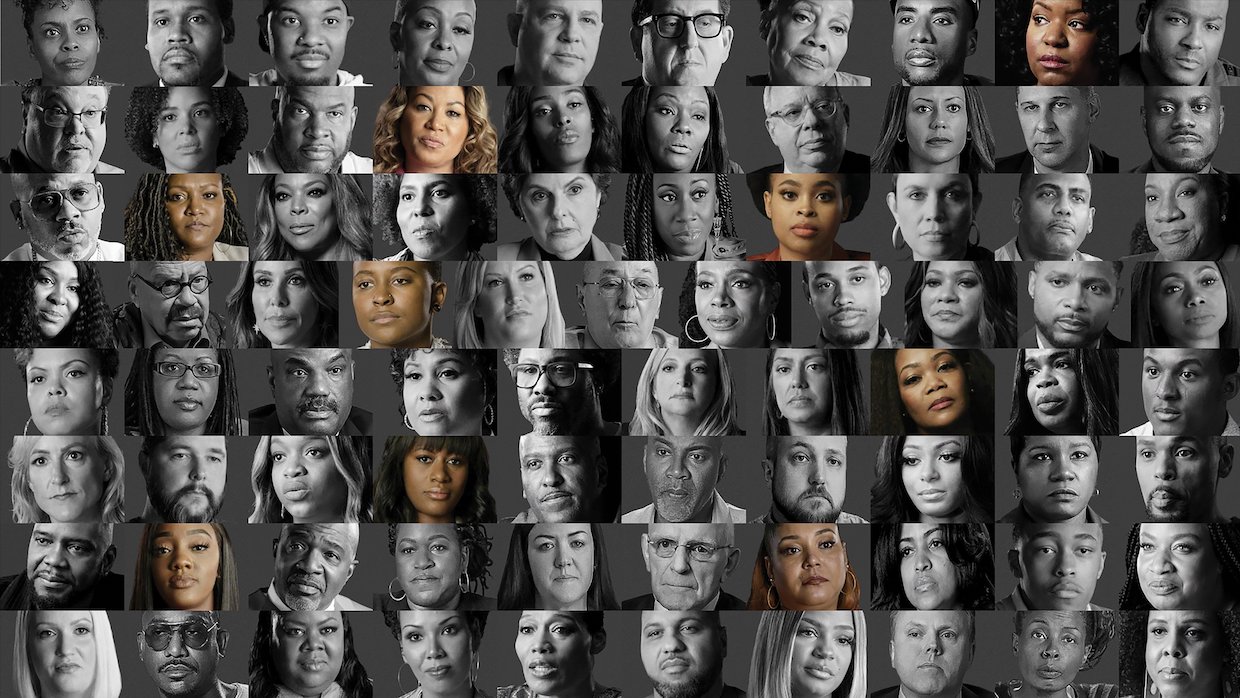This image features a grid of 80 expressive faces, arranged neatly in 8 rows and 10 columns. Each face is displayed within its own square, creating a mosaic-like effect viewed from the front. The majority of these faces are in black and white, enhancing the detail of each expression. However, nine faces are distinctly in color, all of which belong to people of color, suggesting a purposeful inclusion, likely to highlight or signify a specific data point. Recognizable individuals such as C.W. Kamau Bell, Wendy Williams, and Gloria Allred are among the mix. The colored faces are distributed with one in the first row, two in the second, one in the third, one in the fourth, one in the fifth, one in the sixth, and two in the seventh row. The arrangement, while almost perfectly aligned, subtly indicates diversity across gender and race, set against a dark gray background devoid of any text.